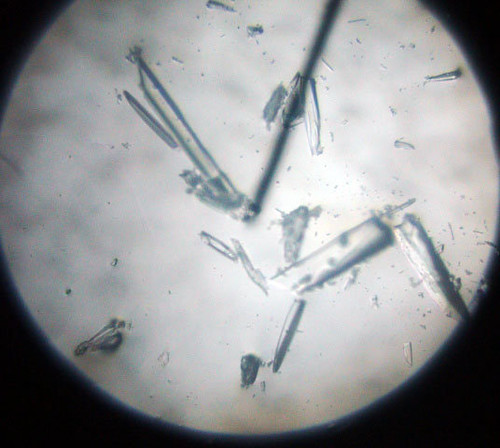This image appears to be a microscope view of a round, whitish-gray, foggy circle that resembles a petri dish. The central area contains a multitude of broken, sharp, crystalline shards. These shards are translucent and vary in shades of gray. Scattered throughout are random gray lines and debris. There are visible fragmented sticks—of which one is notably longer—that seem shattered into tiny bits and pieces. The blurred, murky quality of the image, combined with its smoky appearance, adds to the sense of ambiguity. The outer rim of this lit, grayish-white area transitions to a stark black background, framing the intricate and puzzling scene within.